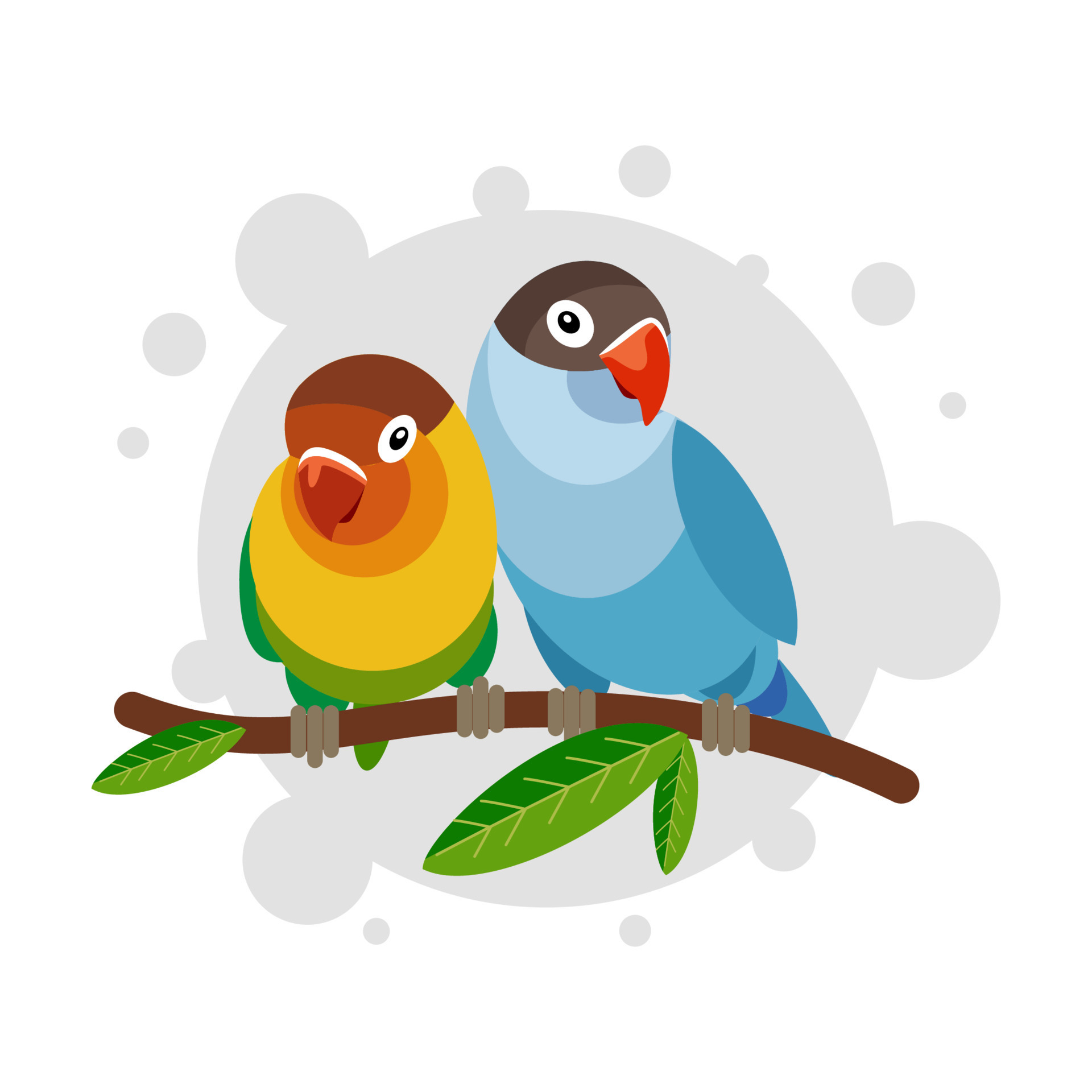This is a colorful and detailed computer-generated cartoon illustration featuring two lovebirds perched on a brown branch with a few pointed green leaves. Set against a clean white background, the birds are enveloped by a large light gray circle, accented by multiple smaller gray bubbles emanating from it. Both birds are presented in a simplistic, one-dimensional style, each with distinct but complimentary coloration, and white eyes with black pupils.

The lovebird on the left is slightly smaller, with a vibrant palette that includes a brown head, a red beak bordered by white, an orange neck fading to a lighter orange, a yellow torso, and green lower body feathers. It has gray feet tightly gripping the branch.

The lovebird on the right is predominantly blue, showcasing various shades that transition from light to dark down its body. It has a grayish-brown head capped with brown and a red-orange beak, also bordered by white. Its feet, similar to the other bird, are gray and firmly wrapped around the branch.

Both birds are leaning slightly towards each other, adding an affectionate touch to the artwork, and appear to be looking in opposite directions. The overall scene exudes a charming and serene atmosphere, capturing the essence of these two tropical birds in a moment of calm companionship.